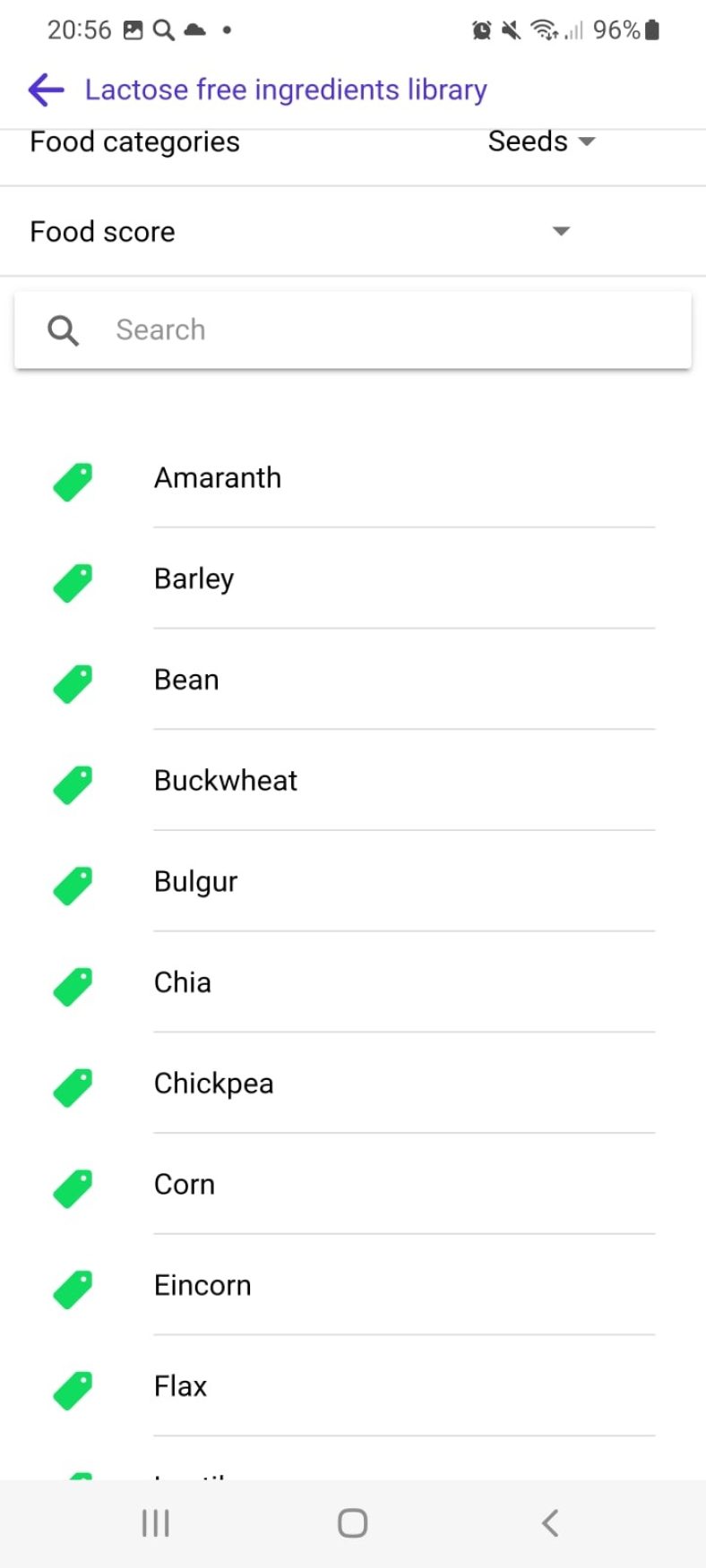This image is a screenshot of a smartphone display, likely running an Android operating system. The time on the device is 20:56, and numerous icons can be seen at the top of the screen: a search icon, a cloud icon, an alarm icon, a mute icon, a Wi-Fi symbol, a cell service indicator, and a battery percentage showing 96%.

The screen content appears to be a webpage or app interface focused on searching for food items, specifically within a lactose-free ingredients library. The title "Lactose-Free Ingredients Library" is displayed in purple font at the top, accompanied by a left-facing arrow icon indicating navigation options.

Below the title, there are two sections: "Food Categories," with "Seeds" currently highlighted, and "Food Score." The screen additionally features a search bar and a vertical list of food items. Each food item is marked with a green tag-like icon on its left side.

The listed food items, in order from top to bottom, are:
1. Amaranth
2. Barley
3. Bean
4. Buckwheat
5. Bulgur
6. Chia
7. Chickpea
8. Corn
9. Einkorn
10. Flax

The final item in the list is partially cut off at the bottom of the screen.

At the very bottom of the screen, there is a navigation bar with three icons: a menu represented by three vertical lines on the left, a rounded square icon in the center (likely the home button), and an arrow pointing to the left on the right side.